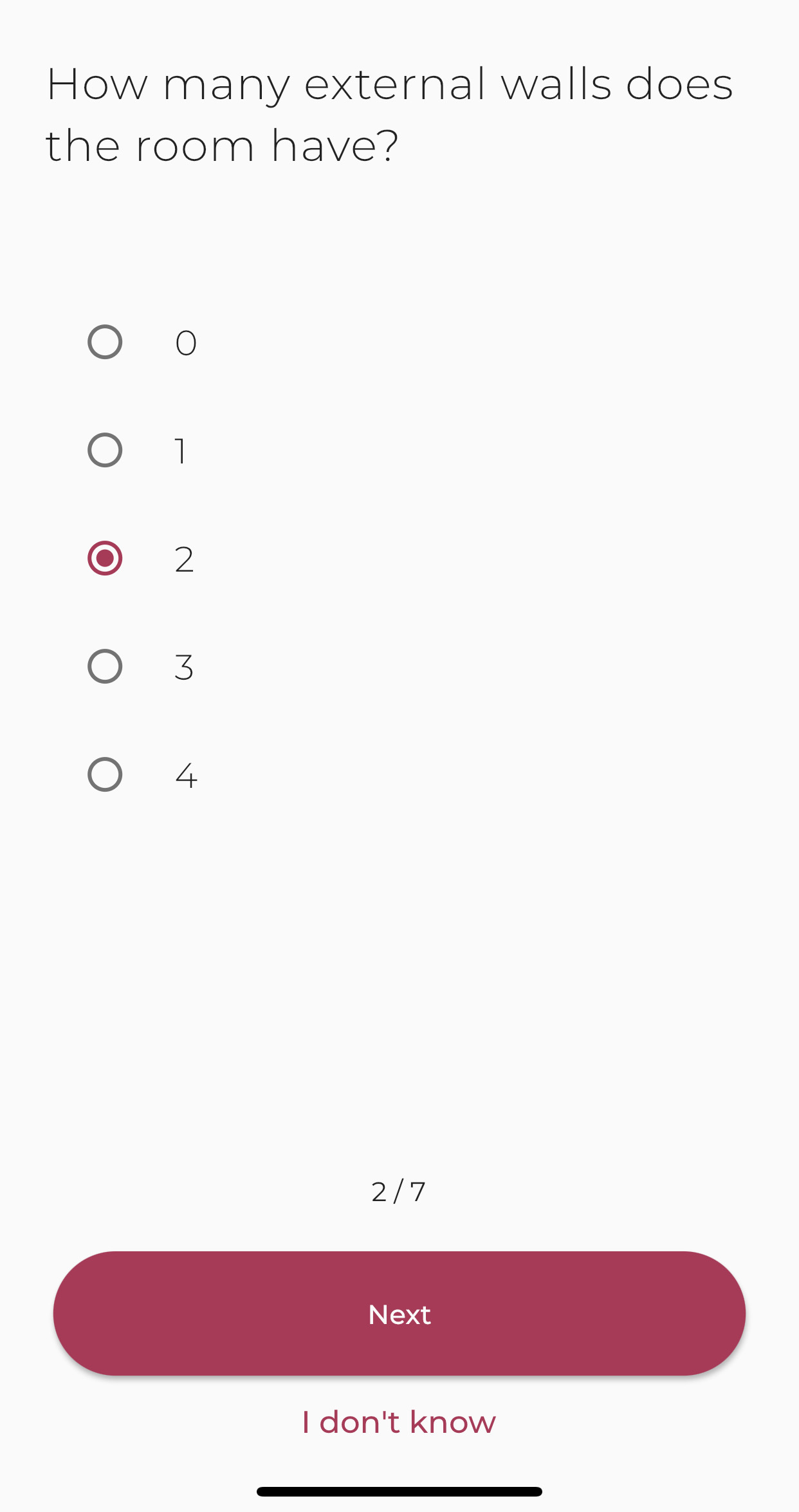A detailed, clean, and descriptive caption for the image:

---

The captured web page is part of a multi-page form, specifically marked as page 2 of 7. The user is tasked with determining the number of external walls for a room, with clickable bubble options ranging from 0 to 4. In this image, the user has selected the option for 2 external walls. 

Navigation options at the bottom of the page include a "Next" button, which is a long, maroon button with squared-off edges, and an "I don't know" button in the same maroon color. Both buttons provide clear guidance for progressing through the form without confusion.

The background of the page is a subtle gray, against which the lighter gray text and numbers are set. Despite their light color, the text and numbers are distinguished enough to remain legible. The absence of a consistent logo or identifiable marker on each page is noted, potentially detracting from a cohesive user experience across the multiple pages.

Overall, the page layout is straightforward, allowing only one selection before proceeding, ensuring clarity in the user's input.